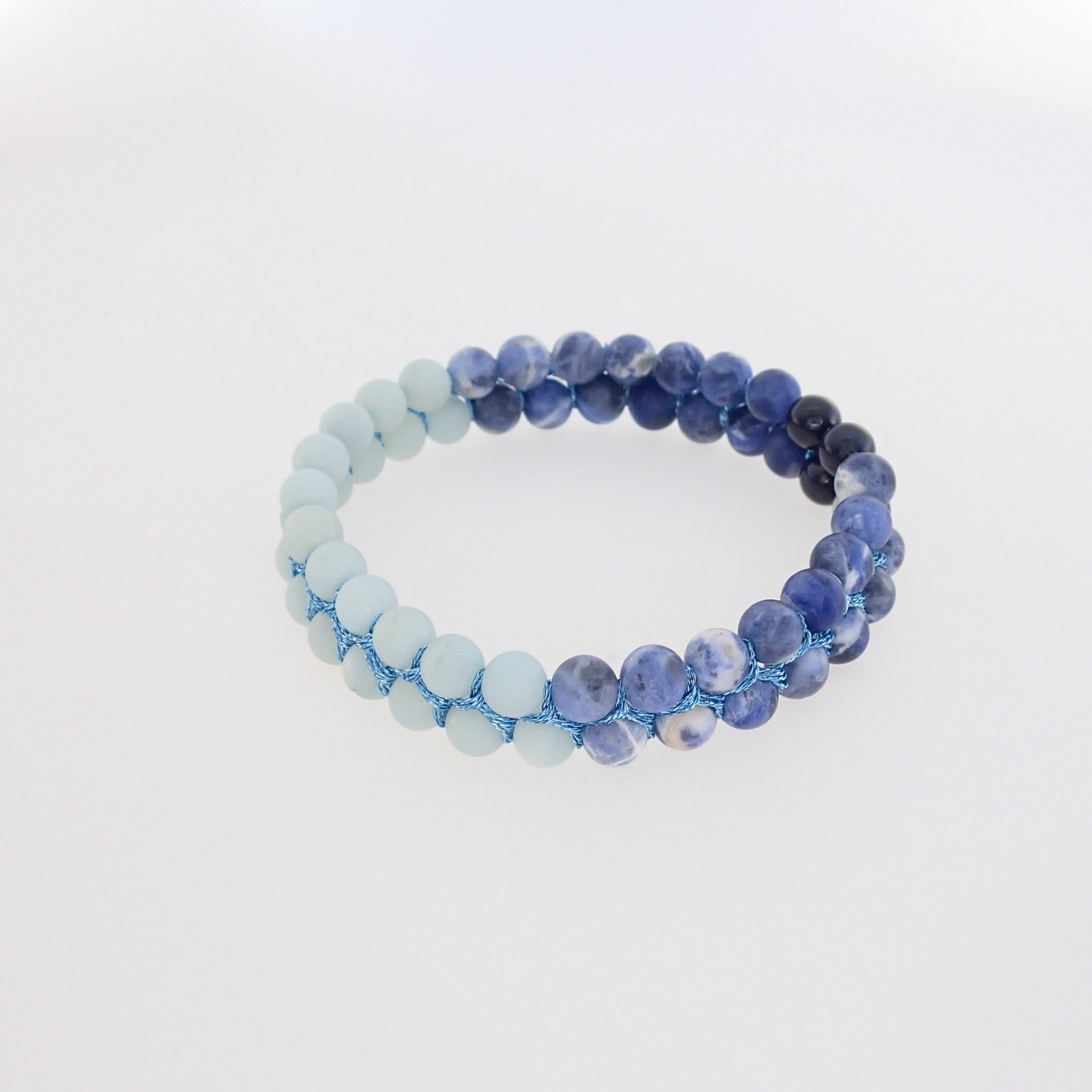This image depicts a close-up, product-style photograph of a multi-colored beaded bracelet set against a plain white background. The bracelet consists of two parallel rows of small spherical beads. The left half of the bracelet showcases white pearl-like beads, while the right half transitions into various shades of blue, with some beads appearing dark blue or even black. The beads are connected by a light blue metallic or wire-like string that adds to the intricate design of the bracelet. The white background is reflective, ensuring full focus is on the detailed craftsmanship of the bracelet.